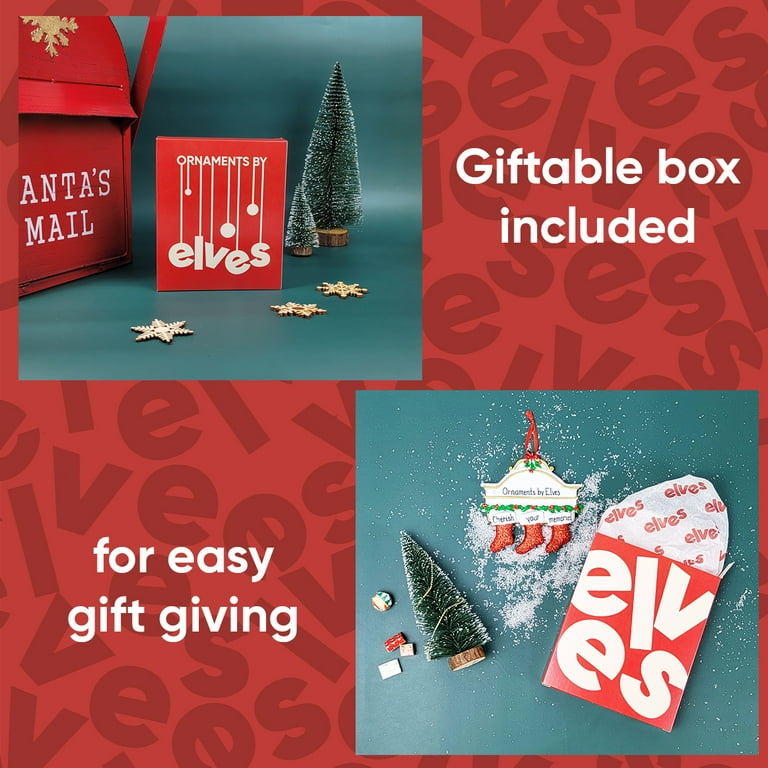The image appears to be an advertisement for "Ornaments by Elves." It is composed of two photographs and several text elements. The background features a red color with darker red text that repeatedly says "Elves" in a large font. In the upper right corner, there is white text stating "Giftable Box Included," while the lower left corner reads "For Easy Gift Giving," also in white. Within the imagery, there are visuals of ornaments, including a tiny Christmas tree and mini stockings that are small enough to fit a thumb. Additionally, the text "Santa's Mail" is partially visible in the upper left, alongside a card that says "Ornaments by Elves" with gold stars at the bottom. The advertisement emphasizes ease of gifting with the inclusion of the giftable box and showcases custom design options for the ornaments, enhancing the Christmas spirit.